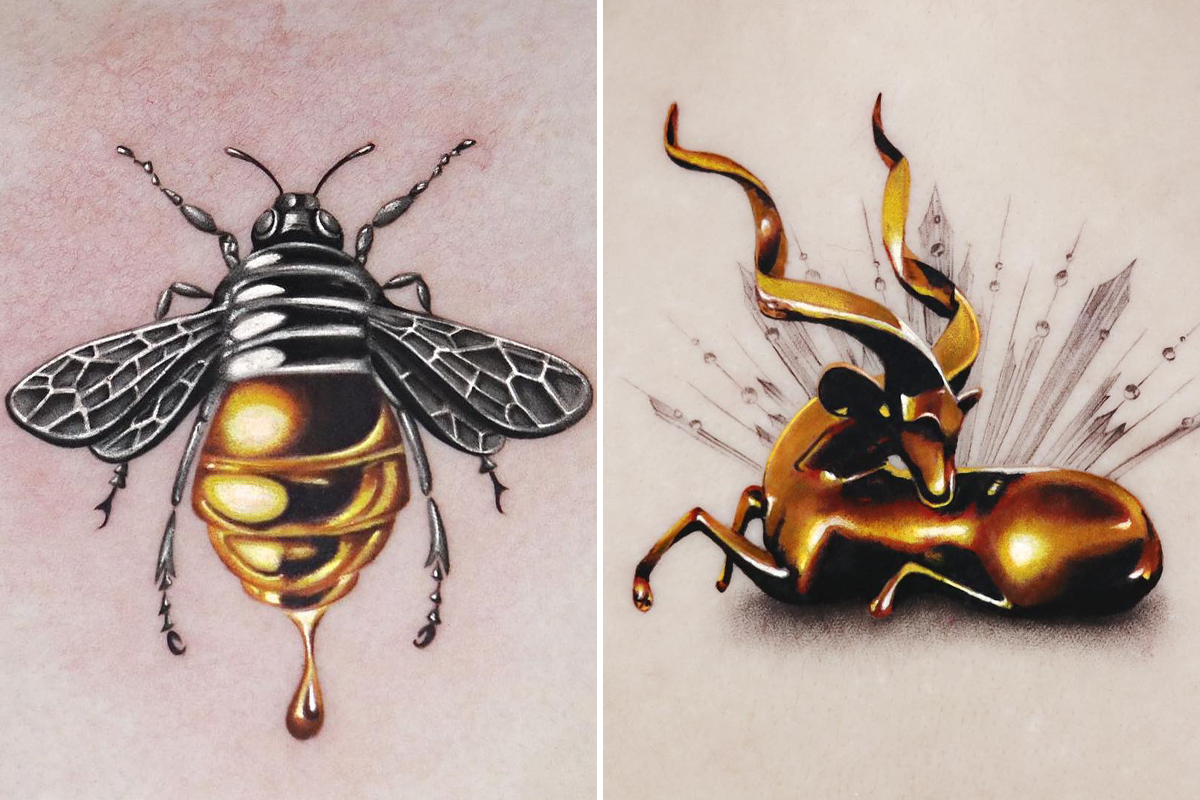The image showcases two side-by-side posters against a pink, marbled background, divided by a thin white vertical line. On the left, there is a highly realistic and lifelike depiction of a honeybee. The bee's abdomen glistens with a metallic, golden shine, accentuated by fluid that drips dramatically, resembling honey, which gives the impression of a textured, 3D effect. The wings and upper body of the bee are designed in black and white, with the wings intricately detailed with silver dividing lines that create a mosaic-like appearance. The legs and antennas are also distinctively black and white, adding to the contrast and intricate design on the person’s skin.

On the right, the poster features a golden deer-like creature with elaborate, spiraling antlers. The animal is captured in a serene, laying position with its legs folded gracefully beneath it. The golden body of the deer is adorned with crystal-like structures that emanate a striking metallic sheen, mirroring the realistic artwork style of the bee. Black lines are artistically drawn behind the deer, forming a burst effect that enhances its majestic and mythical aura. Both images share a consistent style that makes the animals appear metallic and lifelike, leaving a lasting visual impact.